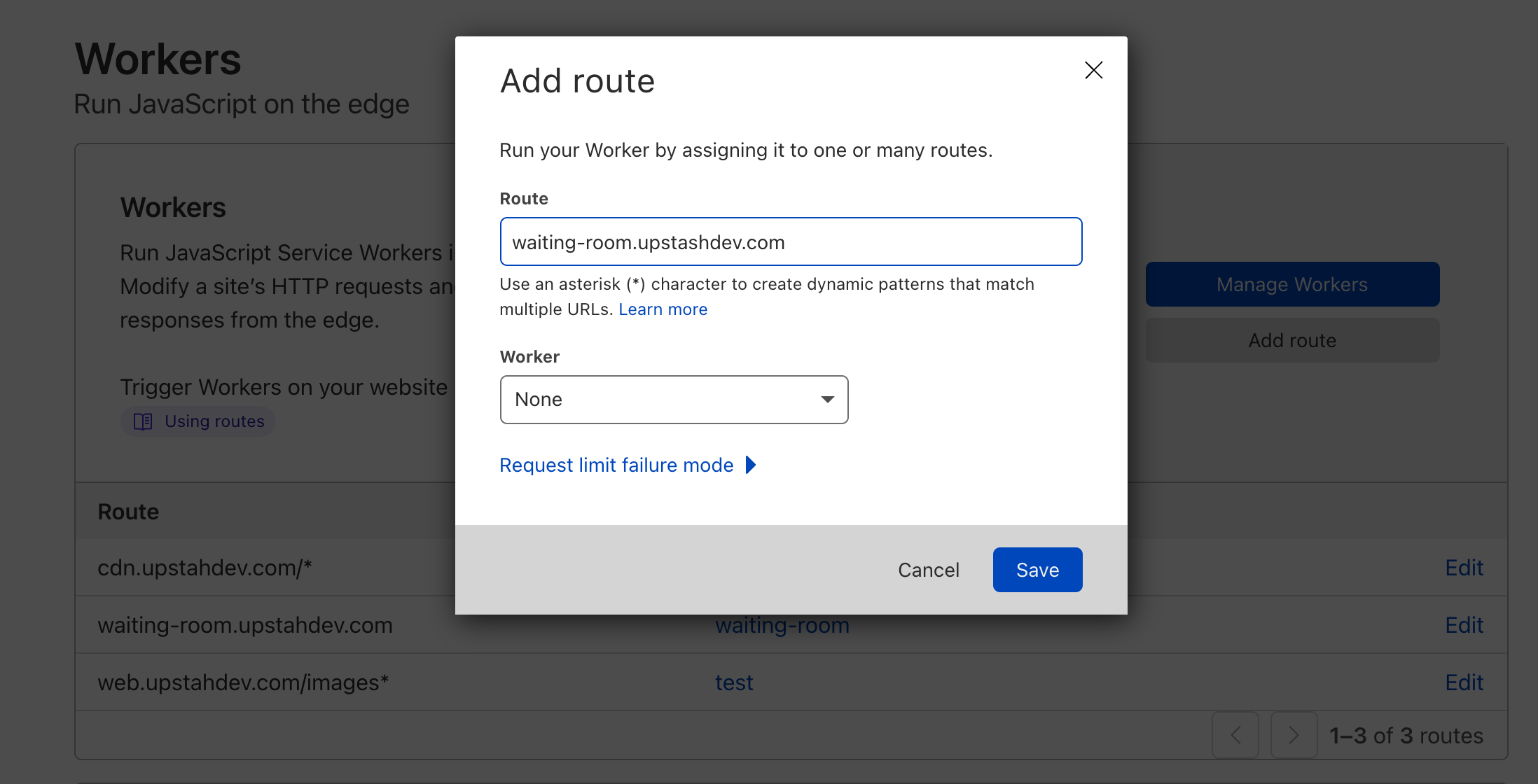In this image, a pop-up window titled "Add Route" is prominently displayed. The pop-up features an 'X' button at the top-right corner for closing the window. The main text of the pop-up reads: "Run your worker by assigning it to one or many routes," followed by examples like "Route: waiting-room.ups or ups-dev.com." It instructs users to use an asterisk (*) character to create dynamic patterns that match multiple URLs. A "Learn More" button is available for further information.

Below this instructional area, there is a drop-down menu labeled "Worker," which currently has "None" selected, allowing users to choose a worker assignment. The pop-up also includes a button labeled "Request Limit Failure Mode." At the bottom of the window, there are two buttons: "Cancel" and "Save."

In the background of the image, the text "Workers run JavaScript on the edge" is partially visible. Additional interactive elements can be seen in the background, such as buttons labeled "Manage Workers" and "Add Route." Some background text is obscured by the pop-up. A section for "Route" displays URL links, including "cdn.ups.dev.com," "waiting-room.ups.dev.com," and "web.ups.dev.com."